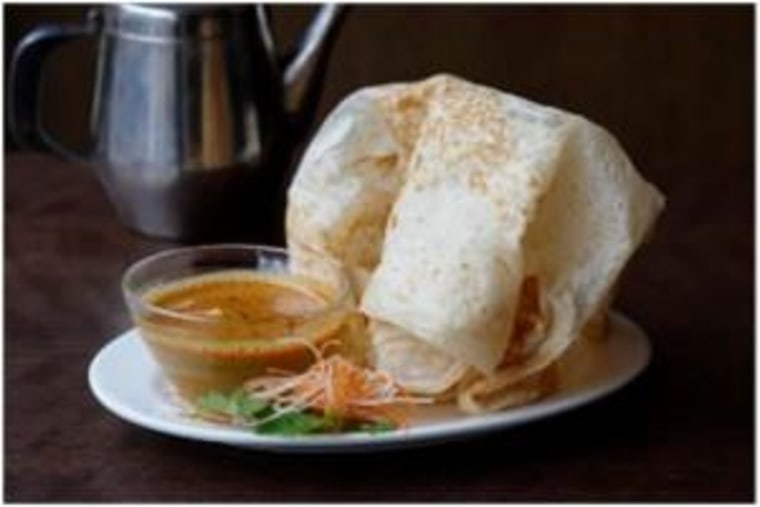The image depicts a close-up, slightly blurry photograph of a plated dish, captured in full color. At the center of the round white glass plate, there is a clear small bowl filled with a dark brown, speckled condiment sauce. Surrounding the bowl, on the left side, are peeled string carrots and some leafy green vegetables. Also featured on the plate is a large, folded cylindrical element that resembles a tortilla but stands tall rather than being wrapped like a burrito. In the background, situated in the upper left corner, is a silver, old-style percolator coffee pot or a stainless steel kettle, indicating an indoor setting, perhaps in a kitchen. The entire arrangement rests on a dark gray dining table, with the right side of the image fading into a dark brown, almost solid, background.